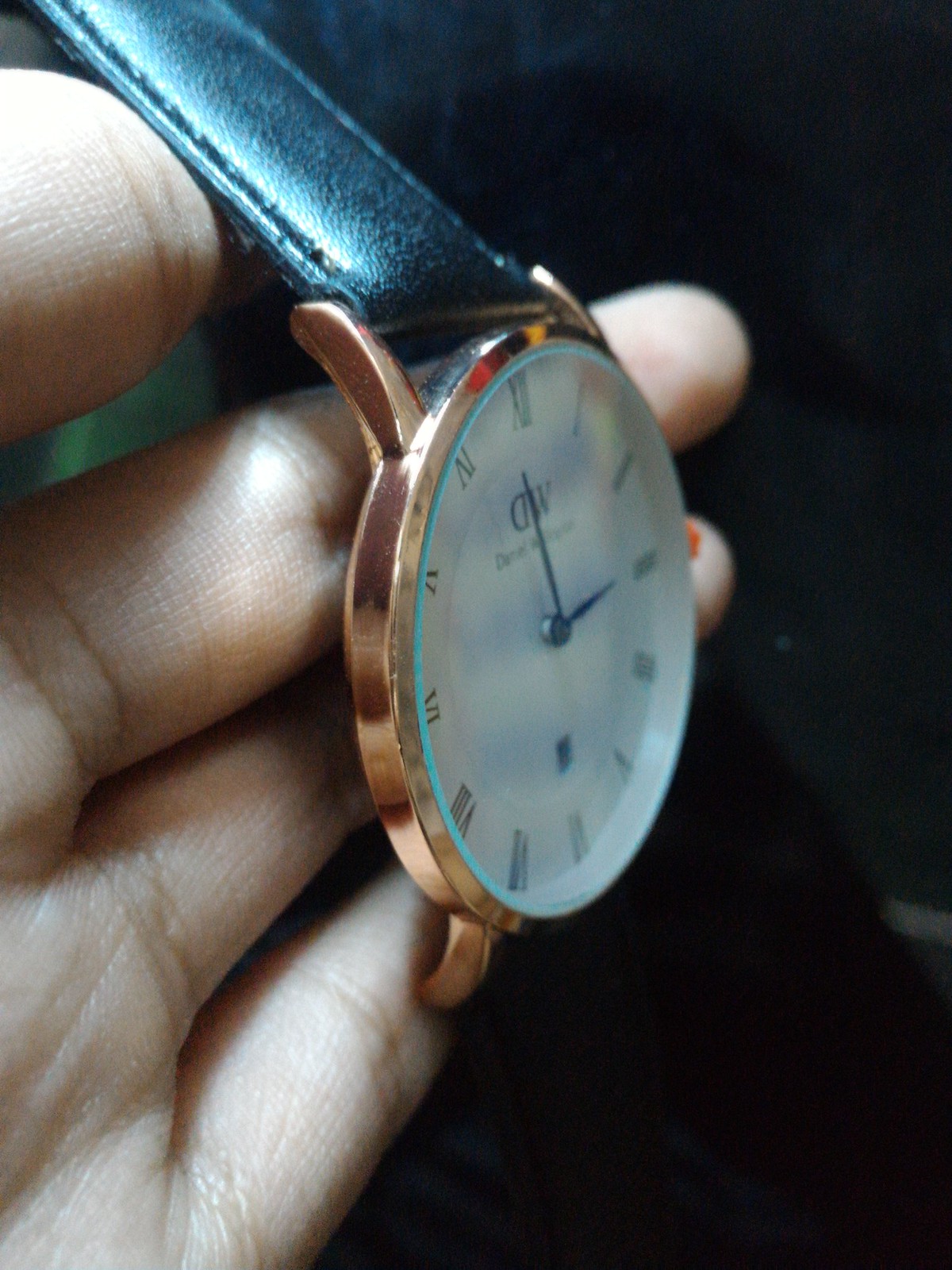This detailed color photograph showcases a classic timepiece resting on the outstretched palm of a hand, likely belonging to a fair-skinned individual. The hand emerges from the left side of the frame, occupying the vertical span from top to bottom, with the watch delicately balanced on the fingers. Only the tips of a couple of fingers are visible on the right edge of the image. 

The watch features a round, white face adorned with black Roman numerals and matching black hands, indicating a time close to three o'clock. Encircling the face is a copper-colored bezel that adds a touch of elegance to the design. The timepiece is further complemented by a black leather band securely attached to the watch body.

The background of the photograph is a solid black, devoid of any discernible details, which accentuates the watch and the hand holding it. Notably, the glass covering the watch face has a blue-tinted edge, reminiscent of a turquoise band, adding a unique and subtle coloration to the overall appearance.